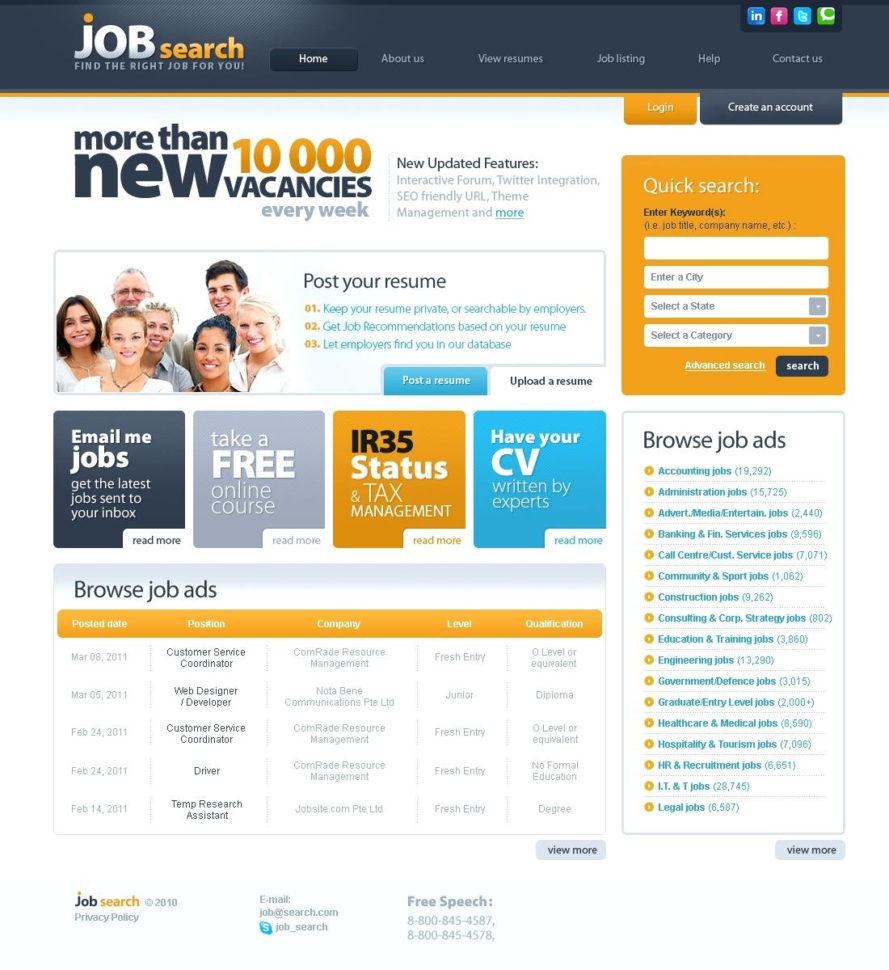Screenshot of a Job Search Website

This screenshot captures a job search website with a structured and user-friendly layout. 

1. **Header:**
   - **Top-left corner**: Features the website's logo with the term "Job Search."
   - **Motto**: Displayed prominently in the header, "Find the right job for you."
   - **Navigation Menu**: Lists sections such as Home, About Us, View Resumes, Job Listings, Help, and Contact Us, all set against a gray background.
   - **Social Media Links**: Located at the very top of the header, above the navigation menu.
   - **User Actions** (towards the right): Options for Login and Create an Account.

2. **Main Content:**
   - **Website Background**: Predominantly white for a clean and professional appearance.
   - **Prominent Banner**: Highlights the website's effectiveness with the text "More than 10,000 new vacancies every week."
   - **Updated Features**: Listed features include an interactive forum, Twitter integration, SEO-friendly URLs, resume management, and more.
   - **Call to Action**: Encourages users to "Post your resume."
   - **Additional Information Links**:
     - "Email me jobs"
     - "Take a free online course" with clickable links for more details.

3. **Job Browsing:**
   - **Browse Job Ads**: Shows a sample list of job advertisements.
   - **Job Categories** (towards the right): Allows browsing based on specific categories such as Accounting Jobs and Administration Jobs.

4. **Search Functionality:**
   - **Quick Search**: Located under the login section, with fields to search by keywords, city, state, and job category.
   - **Advanced Search Option**: Provides a more detailed search functionality.

5. **Footer:**
   - Displays the "Job Search" logo, ensuring branding consistency throughout the page. 

This detailed layout ensures ease of navigation, a variety of search options, and constant updates to meet job seekers' needs effectively.